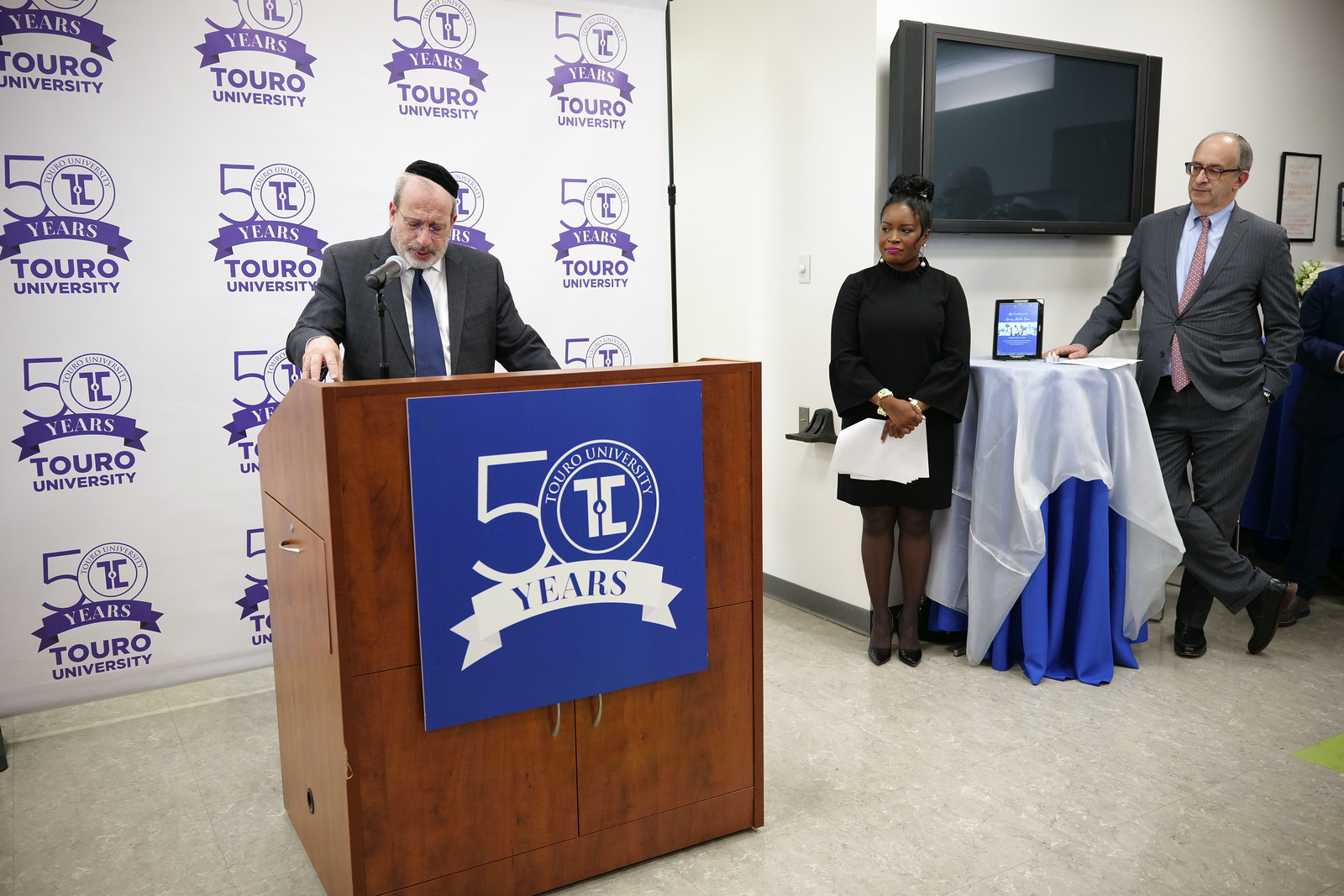The image captures a formal presentation setup featuring a prominent man at a large wooden podium adorned with a blue square logo that reads "50" with "Torino University" inscribed inside the zero. A white banner with blue text below reads "years," celebrating 50 years of Torino University. The man, standing behind the podium, is dressed in a dark gray jacket, a white shirt, and a blue tie. He sports a full beard and a black cap, possibly a yarmulke, and looks down towards the podium, speaking into a microphone. Behind him hangs a white screen displaying "50 years Turo University" in a grid pattern.

To the right of the podium stands a black woman in a black dress, holding white papers in front of her. She has black shoes, her hair styled in a bun, and bright pink lips. Above her, a large CRT TV hangs on the wall over a table draped in both white and blue tablecloths. Next to her, a man in a gray suit with a blue shirt and light pink tie stands with one foot flat on the ground and the other leg crossed, toes touching the ground, gazing towards the left. The atmosphere suggests a commemorative event, possibly honoring 50 years of the university, with all individuals dressed impeccably for the occasion.